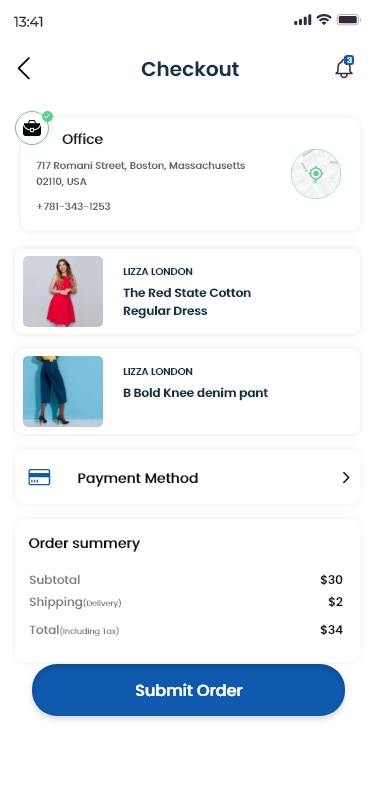This two-panel image depicts a detailed sequence from a cell phone screenshot of an online shopping website. 

**Left Panel:**
- The top portion of the screen displays the current time as 13:41, with indicators for battery life, Wi-Fi strength, and cellular signal strength aligned on the right.
- Just beneath, there's a back arrow pointing left, next to the word "Checkout" written in dark text with a capital "C" centered at the top.
- A notification bell icon appears, showing the number three in white text on a blue background.
- Below the notification, there's a green circle containing a briefcase icon with a checkmark, accompanied by the word "Office."
- Underneath the office label, the address reads: "717 Romani Street, Boston, Massachusetts, 02110, USA," and the phone number is listed as "+781-343-1253."

**First Product Panel:**
- On the left, the product image showcases a girl wearing a sleeveless red dress. 
- The product description above the image reads, "Liza London Red Stage Cotton Regular Dress."

**Second Product Panel:**
- Moving to the right, another product image focuses on a girl's legs, wearing cropped denim pants and black spiked high heels. 
- The description states, "Liza London Be Bold Knee Denim Pant."

**Order Summary:**
- Below the products, the order details are clearly listed:
  - Payment Method: Credit Card
  - Order Summary shows a subtotal of $30, a shipping fee of $2, and a total including tax amounting to $34.
  
**Submit Order:**
- Finally, a blue button with white text invites the user to "Submit Order."

The overall background is largely white, providing a clean and uncluttered look. The left panel captures the structured layout of an online shopping checkout page, with items clearly categorized and labeled for an easy user experience.